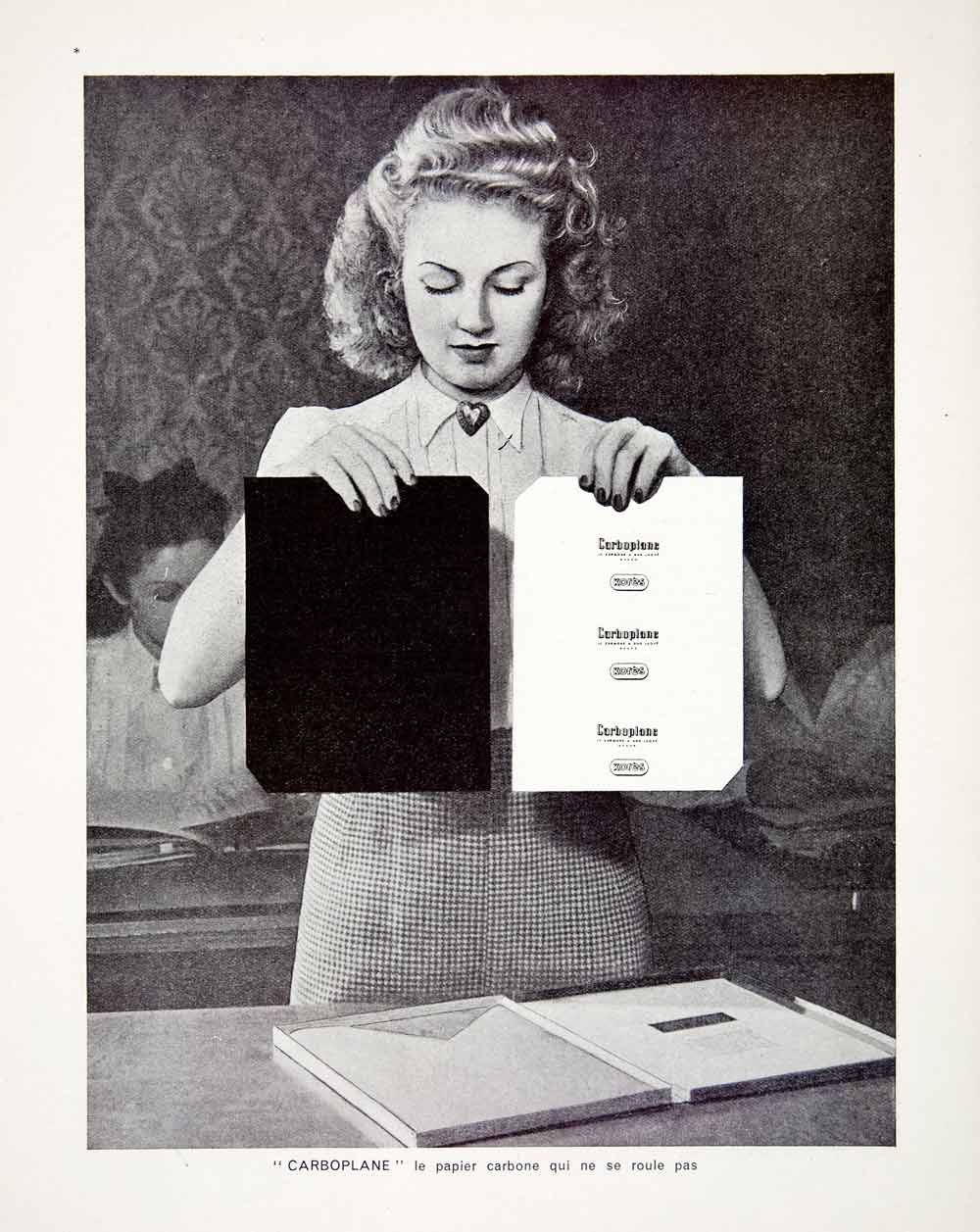This vintage, vertical rectangular black-and-white photograph showcases the charming essence of a bygone era. Encased in an age-yellowed white border, the center of the image features a young Caucasian woman in her 20s with curly blonde hair styled in the fashion of the 1930s. She is dressed in a short-sleeved, collared blouse adorned with a heart brooch at the top of the collar and a plaid herringbone-patterned skirt.

The woman stands in front of a desk, holding two pieces of paper: the one in her left hand is completely black, while the one on her right displays six lines of black text centered on the white paper, though the text is too small to decipher. Her gaze is directed downward at the papers. The desk in front of her contains a writing portfolio with a large envelope on the left and a tablet or pad of paper with a pencil on the right.

In the background, young students are seated at desks, reading books, beneath a vintage-patterned wallpaper. At the bottom of the photograph, there is an illegible caption written in black text along the aged white border. The overall scene, reminiscent of an advertisement, captures a snippet of past daily life with its rich details and nostalgic atmosphere.